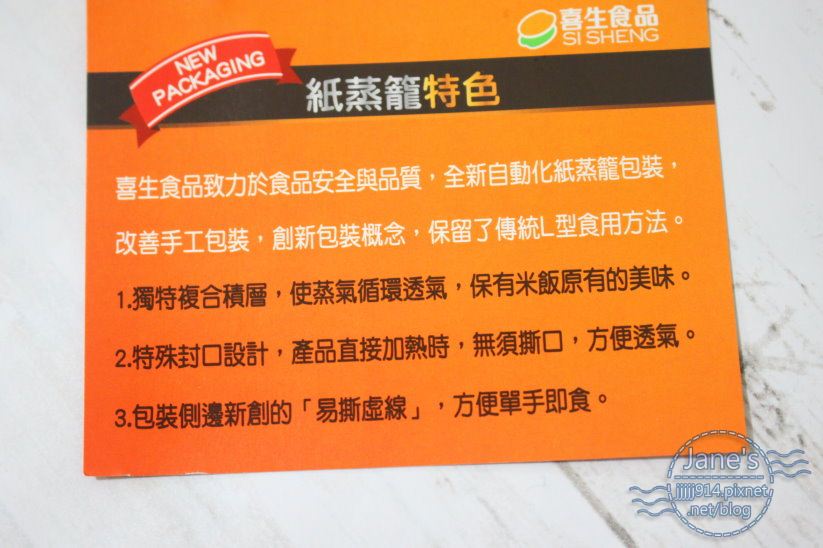The image depicts a rectangular-shaped piece of paper, possibly a business card or flyer, placed on a flat, white marble surface. The background of the paper is predominantly orange, adorned with various Asian characters. At the very top of the paper, a black rectangular strip stretches across with white Asian text. Near the top right corner, there is an orange and green circular logo, and to its left, in white text, it reads "SI Shang." Further down, on the left side, there is a slightly curved red ribbon banner with the white text, "new packaging." At the very bottom right corner is a watermark consisting of a small circle with six wavy lines extending from its sides. Inside the circle, it states "Janes," and below, it lists "JJJJ914.pixnet.net/blog."